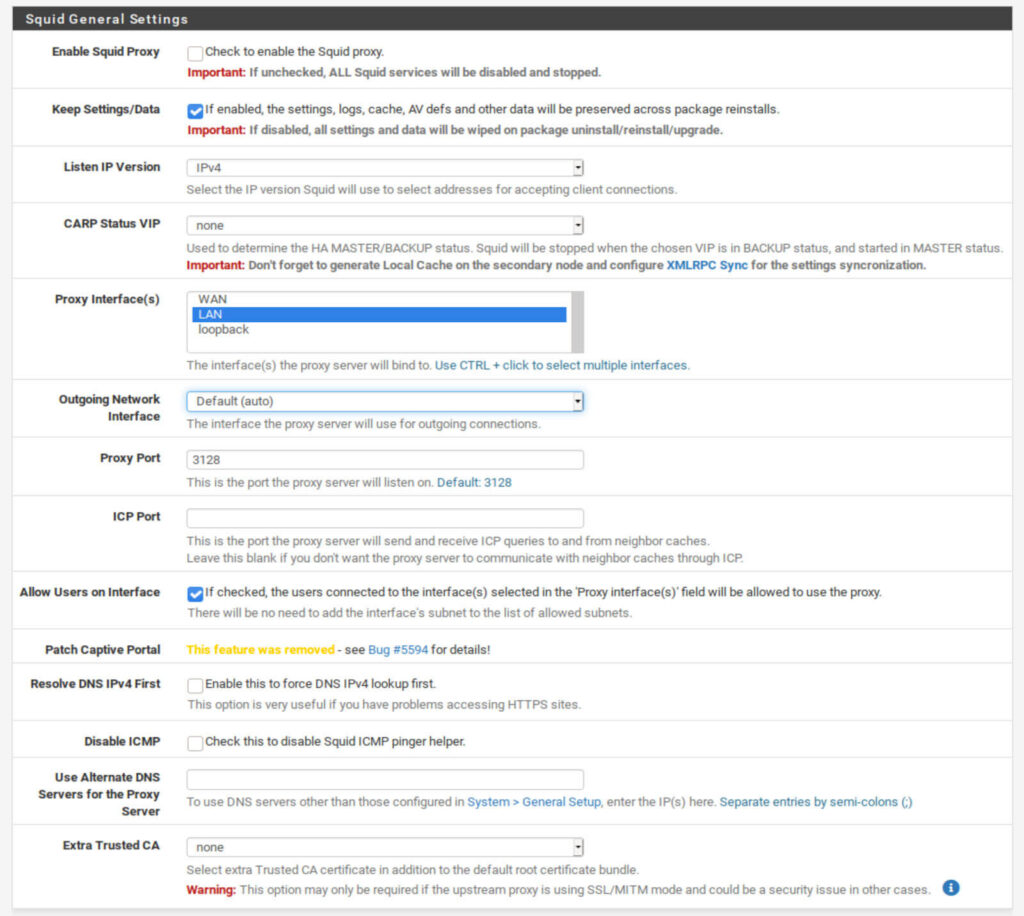The image depicts a settings page from a software interface, likely related to configuring a Squid proxy. The layout includes a thin, light blue border running along the left, right, and bottom edges, while a black border spans the top.

At the top on the left side, in bold white text, it reads "Squid General Settings." Below, on the left side, is a list of settings described in bold text with corresponding settings or input fields to the right.

1. **Enable Squid Proxy**: An empty checkbox next to it.
2. **Important**: In bold red text, followed by a horizontal line.
3. **Keep Settings/Data**: Information displayed to the right.
4. **Listen IP Version**: Information displayed to the right.
5. **CARP Status**: Information displayed to the right.
6. **VIP**: Information displayed to the right.
7. **Proxy Interface**: Information displayed to the right.
8. **Outgoing Network Interface**: Information displayed to the right.
9. **Proxy Port**: Information displayed to the right.
10. **ICP Port**: Information displayed to the right.
11. **Allow Users on Interface**: Information displayed to the right.
12. **Patch Captive Portal**: Information displayed to the right.
13. **Resolve DNS IPv4 First**: Information displayed to the right.
14. **Disable ICMP**: Information displayed to the right.
15. **Use Alternate DNS**: Next line is 
    - **Servers for the Proxy**: Server information to the right.
16. **Extra Trusted CA**: Information displayed to the right.

Gray lines separate each setting to maintain clarity and organization.